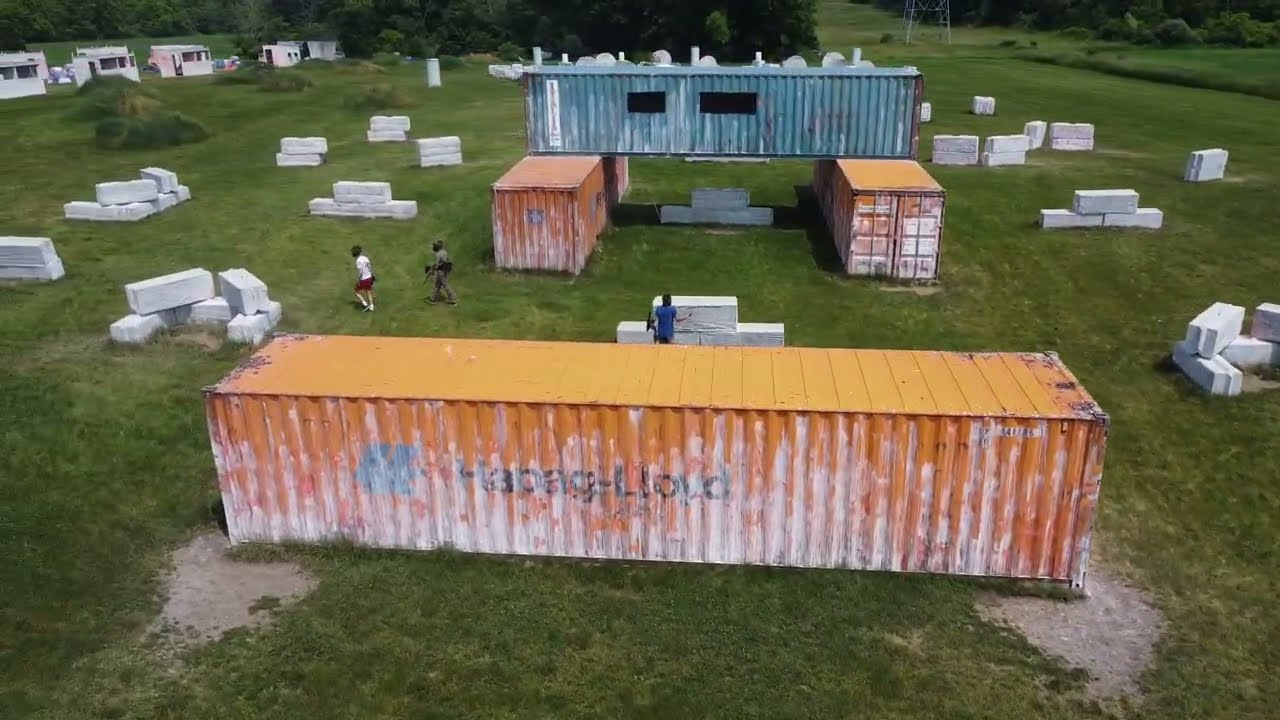This photograph captures a large, grassy open field, scattered with various storage containers. The most prominent feature in the foreground is an orange corrugated shipping container, oriented horizontally, with some kind of blue writing and a blue design on its side, although the specifics are unclear. Directly behind this container, two similar orange containers stand upright, perpendicular to the first. Bridging across these vertical containers is a large blue corrugated container, laying horizontally, notable for its two visible rectangular windows.

The field is dotted with numerous white storage containers, each about six or seven feet long, based on their scale relative to the people nearby. These white containers are arranged in different stacks and piles throughout the area. Particularly, some white containers are clustered just beyond the central orange container, with a person standing beside them, and others are scattered on the left and right sides of the image.

In the middle background, beneath the blue container, several white containers can also be seen. Three people are visible within the scene: one appears to be partially hidden behind a container, while two others are seen walking on the left side of the photo. In the upper left-hand corner of the background, a row of small buildings, three or four in number, is discernible.